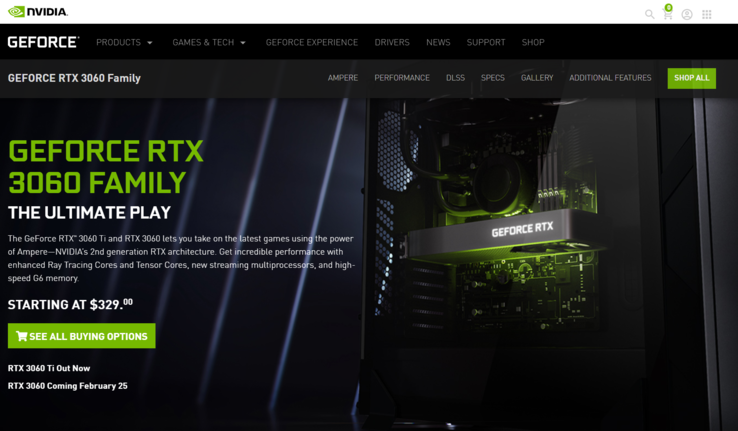The image depicts a screenshot of the NVIDIA website, with proportions approximately twice as wide as it is tall. At the top of the image, a white navigation bar spans the full width, occupying about 5-10% of the vertical space. The top-left corner of this bar features the NVIDIA logo, showcasing the distinctive green swirl followed by the text "NVIDIA."

The top-right corner of the white bar displays several navigation icons: a search icon, a shopping cart, a user profile icon, and a 3x3 grid of dots, suggestive of additional options or applications.

Beneath the white navigation bar, the background transitions to a predominantly black or gray hue, marking the beginning of the menu section. On the left side of this section, in bold white text, the title "GeForce RTX 3060 Family" is prominently displayed. Aligned to the right are the navigation links, listed in gray text: "Ampere," "Performance," "DLSS," "Specs," "Gallery," and "Additional Features." At the far right is a green button, styled in NVIDIA's signature GeForce green, with the label "Shop All" in white text.

Lower down, the main banner area is highlighted, featuring a detailed right-side view of a PC case. The interior of the case is visible, prominently displaying a GeForce RTX graphics card. The top of the graphics card emits a green light that illuminates the surroundings and the motherboard beneath it, casting a striking visual effect.